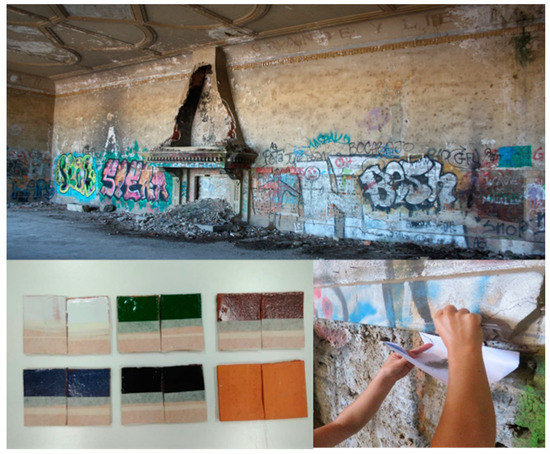The image consists of three photos that collectively depict an abandoned mansion room with elaborate ceiling designs and a fireplace, overlaid with colorful graffiti. The main wall, adorned in bright graffiti with colors like black, white, aqua, yellow, pink, and purple, contrasts starkly with the room’s otherwise neutral tones of black, white, orange, and tan. Beneath this vibrant display, a photograph on the bottom left showcases an array of colored rectangles that resemble paint samples or possibly glazed tiles in hues of white, green, maroon, navy, black, and orange. The lower right image features a close-up of two arms and hands, which appear to be in the process of removing or scratching at the graffiti on the wall. The abandoned room, highlighted by ornate ceilings and graffiti-covered walls, has an air of neglect and creative defacement, with the various elements from each photo coming together to tell a story of decay and attempted restoration.